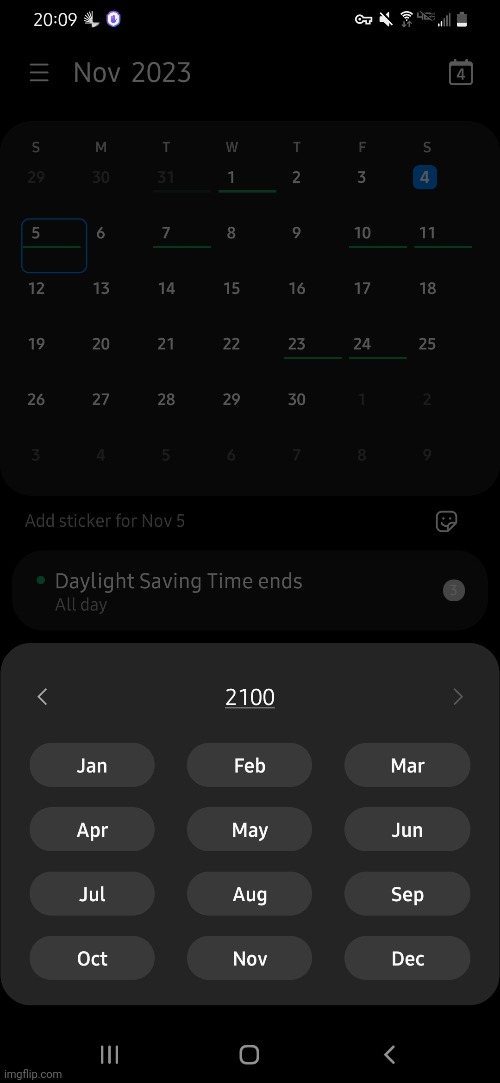This image is a screenshot from a Samsung phone's calendar app, featuring a dark theme with a black background. At the top of the screen, the status bar displays the current time on the left side, alongside various icons such as no alerts, Wi-Fi, and battery status on the right.

The calendar is open to the month view for November 2023. The date "November 4" is highlighted, suggesting that today’s date is November 4th. Several dates within the month display small bars, indicating scheduled events or reminders on those days. Below the calendar grid, there's a text prompt reading "Add sticker for November 5," followed by a reminder note, "Daylight Saving Time ends," labeled as an "All day" event.

A secondary window at the bottom shows a broader timeline with all months from January to December for the year 2100, hinting at a feature to navigate through years quickly. The image also includes the standard navigation buttons at the bottom: "All Tabs," "Home," and "Back."